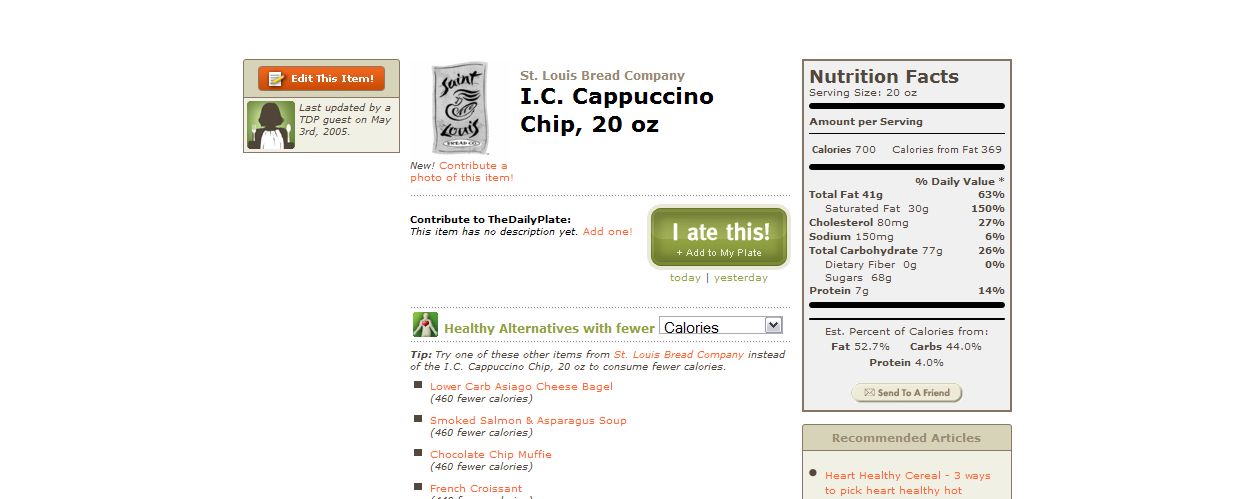The image displays detailed nutritional information for a product from the St. Louis Bread Company, specifically an I.C. Cappuccino Chip, 20 oz. In the upper left-hand corner, there is a small box with a notation: "Edit this item last updated by a TDP guest on May 3rd, 2005." The box also features a gray logo with "St. Louis" emblazoned on it. 

Below this, the product's title is prominently stated as "St. Louis Bread Company, I.C. Cappuccino Chip, 20 oz." Accompanying this title are prompts inviting users to contribute a photo of this item or add it to their daily meal tracker. It suggests users can log that they ate it today or yesterday. Additionally, it offers suggestions for healthier alternatives with fewer calories, such as a lower-carb Asiago cheese bagel, smoked salmon asparagus soup, a chocolate chip muffin, and a French croissant.

The central focus of the image is the nutritional facts section. It lists the following details: 
- **Serving Size**: 20 oz
- **Calories**: 700
- **Calories from Fat**: 369
- **Total Fat**: 41 g
- **Saturated Fat**: 30 g
- **Cholesterol**: 80 mg
- **Sodium**: 150 mg
- **Total Carbohydrate**: 77 g
- **Dietary Fiber**: 0 g
- **Sugar**: 68 g
- **Protein**: 7 g